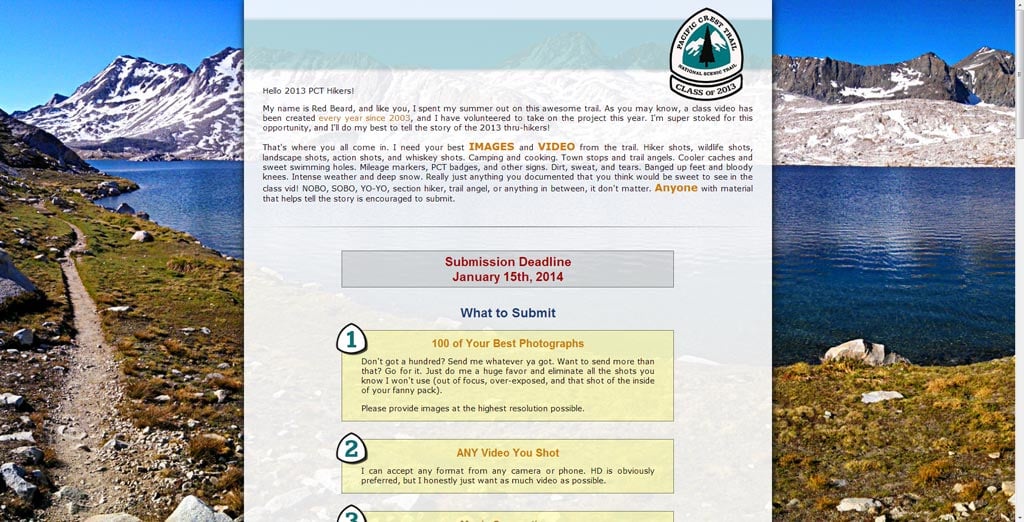A captivating banner advertisement featuring breathtaking natural landscapes with a call for submissions. On the left side, the image showcases a serene nature area adjacent to a pristine, deep blue lake, flanked by snow-covered rocky outcrops. On the right side, another picturesque scene displays vibrant greenery and rugged walking trails amidst rocky terrain. Above these images, set against a clear, blue sky, the banner reads "Pacific Crest Trail," adorned with a symbolic patch. The center prominently displays a heartfelt message to the "Class of 2013 PCT hikers" from someone known as Red Beard. He recounts his unforgettable summer on this trail and invites fellow hikers to contribute their memories. Participants are encouraged to submit 150 of their best photographs or videos by January 15, 2014, for a commemorative project. The banner eloquently balances the natural beauty of the trail with a personal and engaging call to action, inspiring the community to share their experiences.